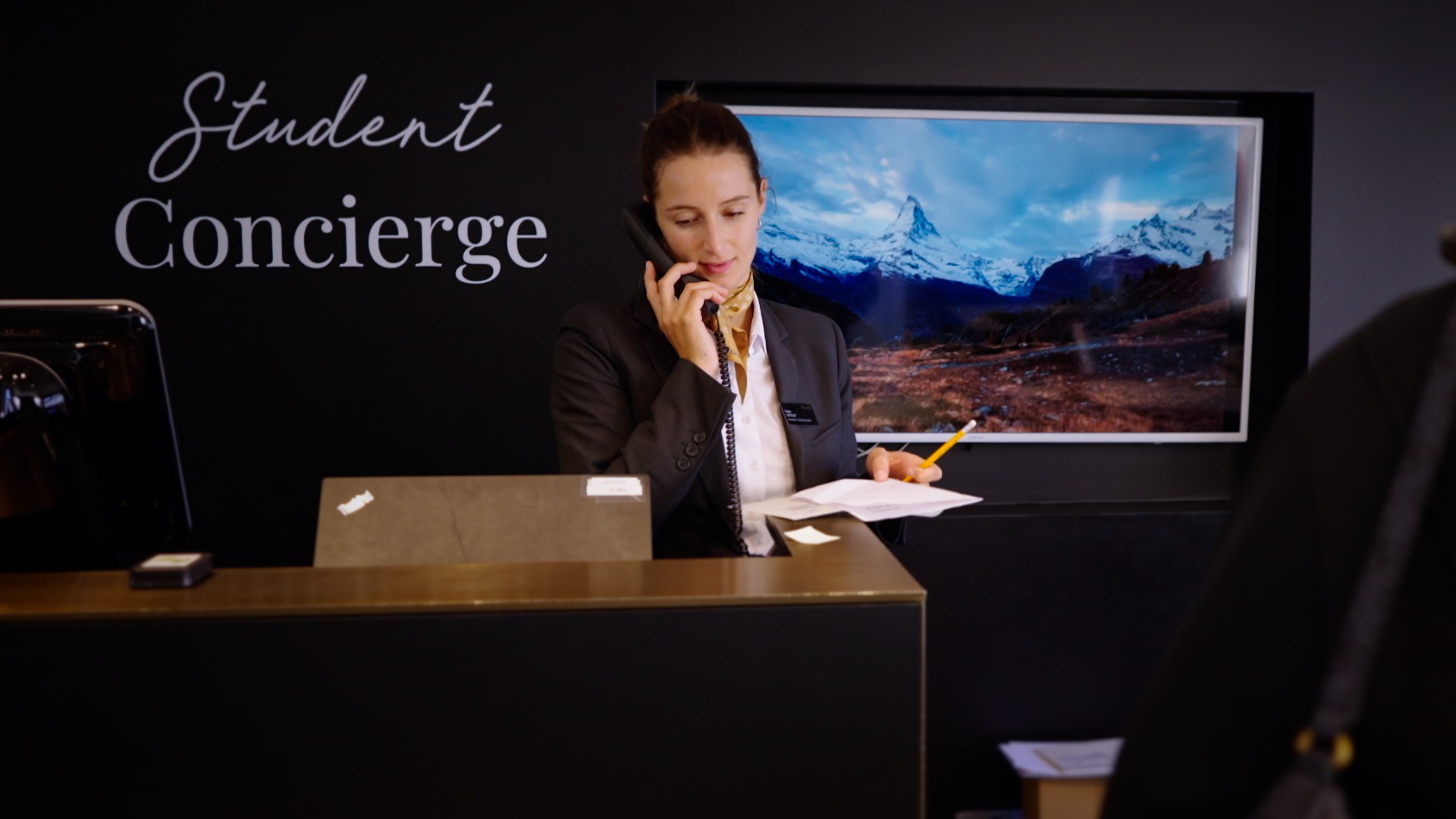A professional woman with her black hair neatly styled in a bun sits at a desk, engaged in a phone conversation using a corded phone held in her right hand. Clad in a sophisticated black suit and white shirt, she appears focused, slightly smiling, and looking down at a piece of paper in front of her on the desk, with a pencil in her left hand. The desk is a mix of brown and black hues. 

Behind her, a wall bearing the white text "Student Concierge" is visible on a black background. To her left, a monitor or a picture displays a scenic view of snow-capped mountains under a blue sky with some grass and brown dirt in the foreground. Additionally, the edge of another person carrying a bag or piece of luggage is just visible in the frame. Further on the desk, there's a ThinkPad laptop along with another electronic device, likely used for credit card payments, enhancing the professional and service-oriented setting.